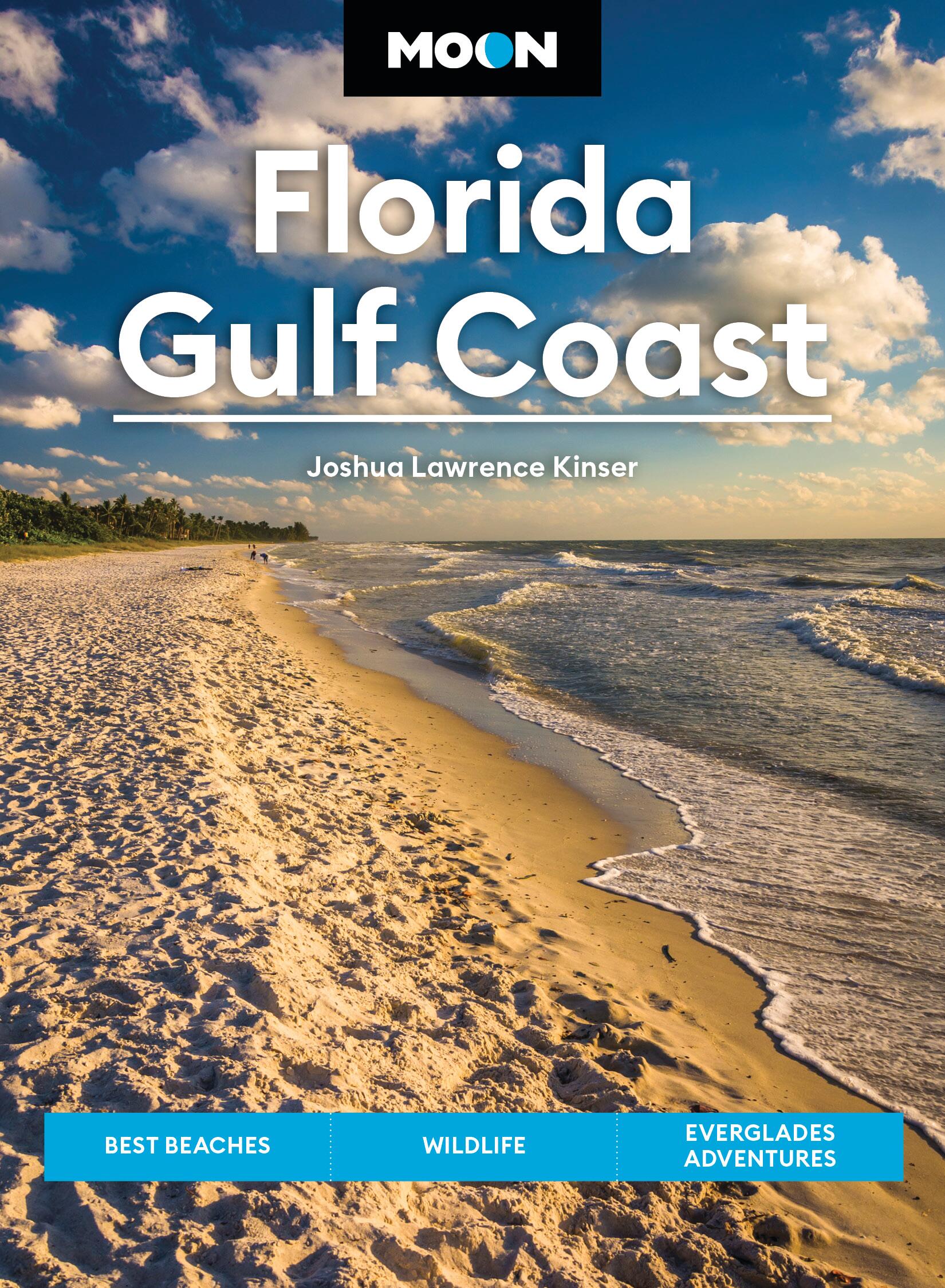The cover of this guidebook, titled "Florida Gulf Coast" by Joshua Lawrence Kinzer, is a vibrant and inviting portrayal of a quintessential Florida beach. The publisher's logo, "Moon," appears at the top center in a one-inch wide black rectangle with white text; the second "O" is uniquely styled with a turquoise circle and a white crescent. The top two-fifths of the cover showcases a clear blue sky adorned with fluffy white clouds, while the bottom depicts a serene beachscape. The left side of the image is dominated by beige sand covered in numerous footprints, and gentle, white-capped waves lap up against the shore from the brackish gray ocean on the right. Overlaying this picturesque scene, near the bottom, is a bold blue rectangle containing white text that reads "Best Beaches, Wildlife, and Everglades Adventures." Additionally, the title "Florida Gulf Coast" appears prominently in large white font, with "Gulf Coast" underlined by a white horizontal bar, and the author's name, "Joshua Lawrence Kinzer," is inscribed beneath it in smaller print.